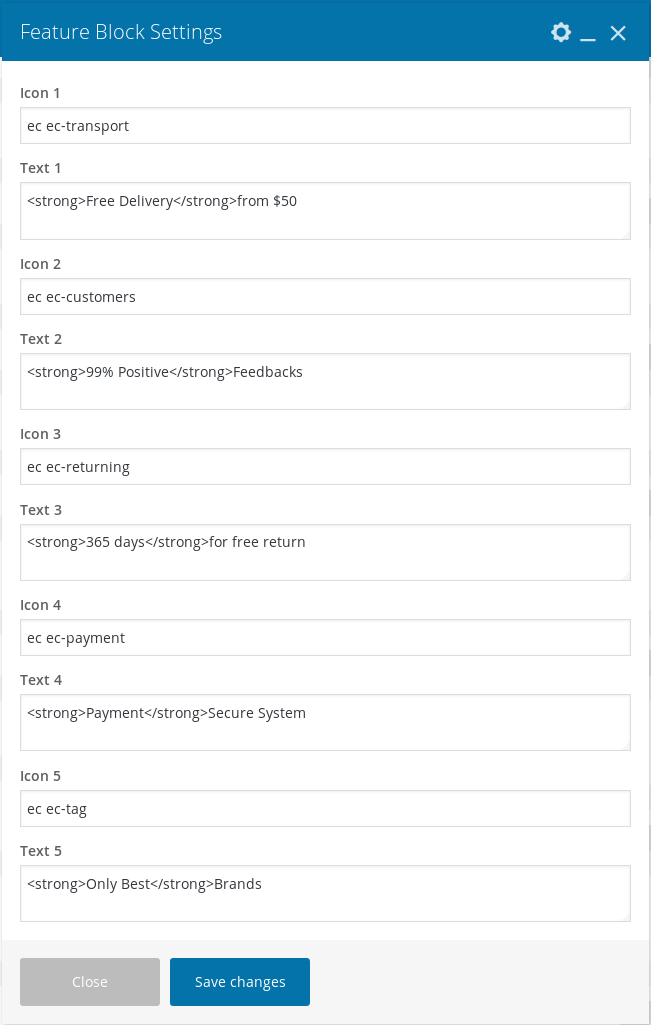This digital image showcases feature block settings, consisting of five distinct sections, each depicting unique services accompanied by respective icons and descriptive texts:

1. **Icon 1: EC Transport**
   - **Text 1:** **Free delivery**. Available **from $50**.

2. **Icon 2: EC Customers**
   - **Text 2:** **99% positive** feedback from our valued customers.

3. **Icon 3: EC Returning**
   - **Text 3:** **365 days** for **free return** policy.

4. **Icon 4: EC Payments**
   - **Text 4:** **Payment** methods are protected by a **secure system**.

5. **Icon 5: EC Tag**
   - **Text 5:** **Only the best** brands available.

Additionally, the interface features a gray-colored "Close" button and a blue-colored "Save Changes" button for user interaction.